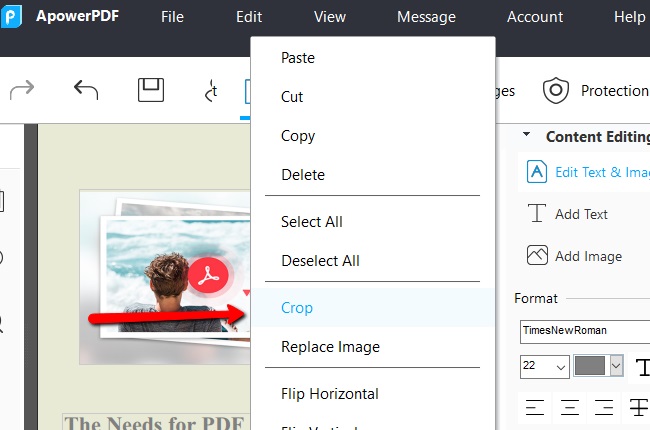The image displays a detailed screenshot from a website interface, specifically from a PDF editing software. 

At the very top, there is a black navigation bar approximately an inch thick, spanning the entire width of the screen. Within this bar, on the left-hand side, there is a white box with the letter "P" enclosed. Next to this, in white text, it reads "A Power PDF." Following this, the menu options, all in white text, include "File," "Edit," "View," "Message," "Account," and "Help," aligned horizontally.

Beneath the black navigation bar, in the top-left corner, there are two arrow icons—a gray one that bends left after pointing upwards and a black one similarly shaped. Adjacent to these arrows is an icon representing a floppy disk, followed by an icon of a lowercase 't' with a distorted black line resembling a 'C' on its left.

Next in line is a pop-up menu listing several text editing options in black: "Paste," "Cut," "Copy," and "Delete," each separated by a standard black line. Below these options are "Select All" and "Deselect All," also divided by a black line. The "Crop" option is distinguished in blue with a lighter blue highlight. Following this, options revert to black text—"Replace Image," segmented by another black line, then "Flip Horizontal."

On the right side of the main interface, immediately under the black bar, is an icon of a black shield with an outlined black circle inside it. To the right of this icon, it says "Protection" in black, followed by "Content Editing." Below this text, a white box with a blue 'A' appears, highlighted in blue, with the accompanying text "Edit Text & MIMA" in blue. Underneath, another icon with a black 'T' signifies "Add Text," and right below that, a black outlined box with two mountains inside signifies "Add Image." Below this is another text header, "Format."

Adjacent to this section, towards the right edge of the image, is a white box outlined in black labeled "Times New Roman," followed by a drop-down menu labeled "Choo Choo." Alongside this is another white box containing a black bar within it and an additional drop-down menu. Immediately to its right is a 'T' icon, followed by three alignment options depicted as three lines in varying positions, and lastly, another 'T' icon with a black line striking through it.

Underneath the initial pop-up menu and further down the page, there is a beige-colored background featuring an image of a figure with short brownish hair wearing a gray T-shirt, facing away from the camera and looking out towards an ocean. Below this image, in gray text, it reads, "The Needs for PDF."